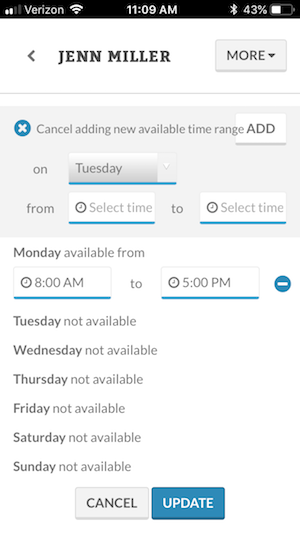The image displays a screenshot with various interface elements, each providing specific information. In the top-right corner, a battery icon indicates a 43% charge, displaying a half-full white color. Adjacent to the battery icon, a Bluetooth icon is also visible, colored in white. In the center of the top section, the current time is shown as 11:00 AM. To the left of the time, the Wi-Fi signal strength icon indicates full bars. Following that, the word "Verizon" appears next to a signal strength icon showing 2 out of 4 bars.

In the top middle of the image, the name "Jen Miller" is displayed with a left-pointing arrow next to it. To the right of the name, inside a boxed area, is the word "More" with a downward arrow. Below a thin horizontal line, there's another boxed area containing the phrase "Cancel adding new available time range." The text below this specifies the availability on Tuesday with two boxes labeled "Select time" indicating the start and end times to be chosen.

Further down, the words "Monday available from" are shown, with two boxes beneath them. The left box shows "8 AM" and the right box shows "5 PM." Adjacent to the "5 PM" box, there's a circle featuring a white rectangular bar. This detailed time selection interface is situated in the middle of the screenshot.